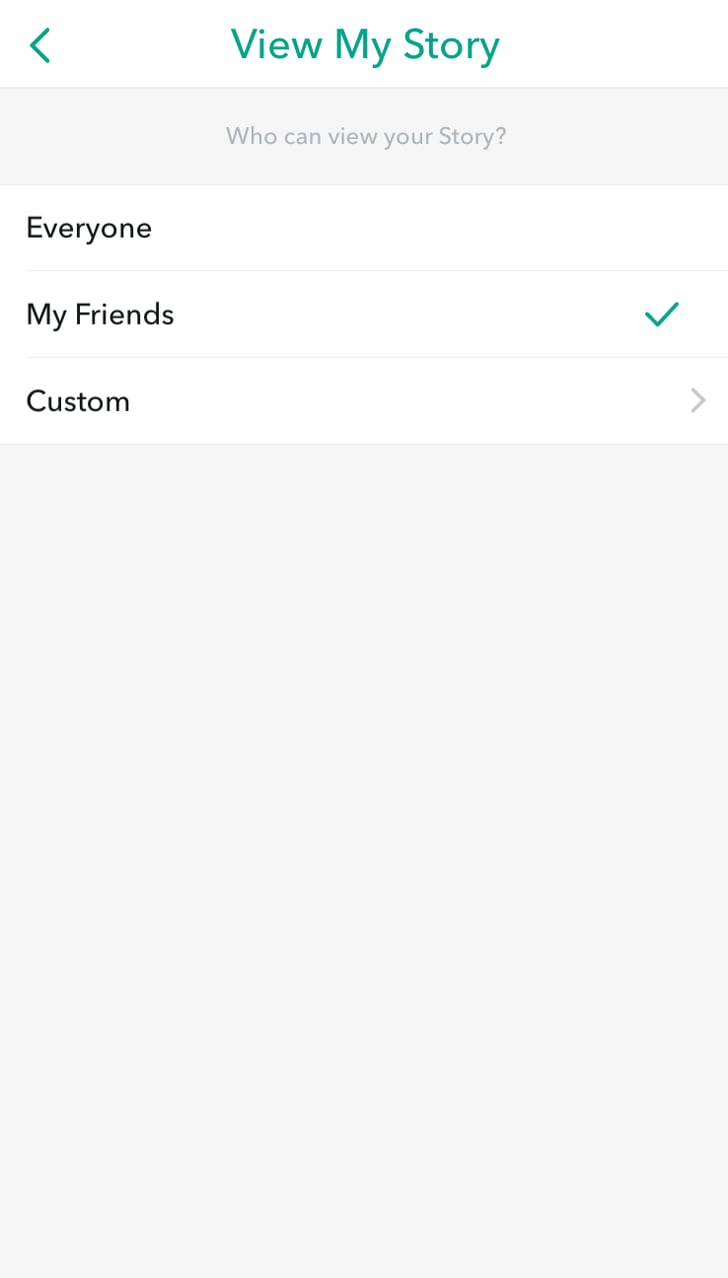The image showcases a settings page from WhatsApp, allowing the user to customize who can view their story. At the very top, there is green text reading "View My Story," centered against a white background. On the top left corner of the image, there is a green back button. Below the "View My Story" header, smaller gray text on a light gray background reads, "Who can view your story."

Three selectable options are listed under this prompt, each against a white background with black text. The first option reads "Everyone," the second "My Friends," and the third "Custom," which has a gray arrow icon pointing to the right, indicating it’s a selectable option with further settings. The option "My Friends" is currently selected, marked by a green checkmark on its right side. The background of the image is a light gray, consistent with the WhatsApp theme.